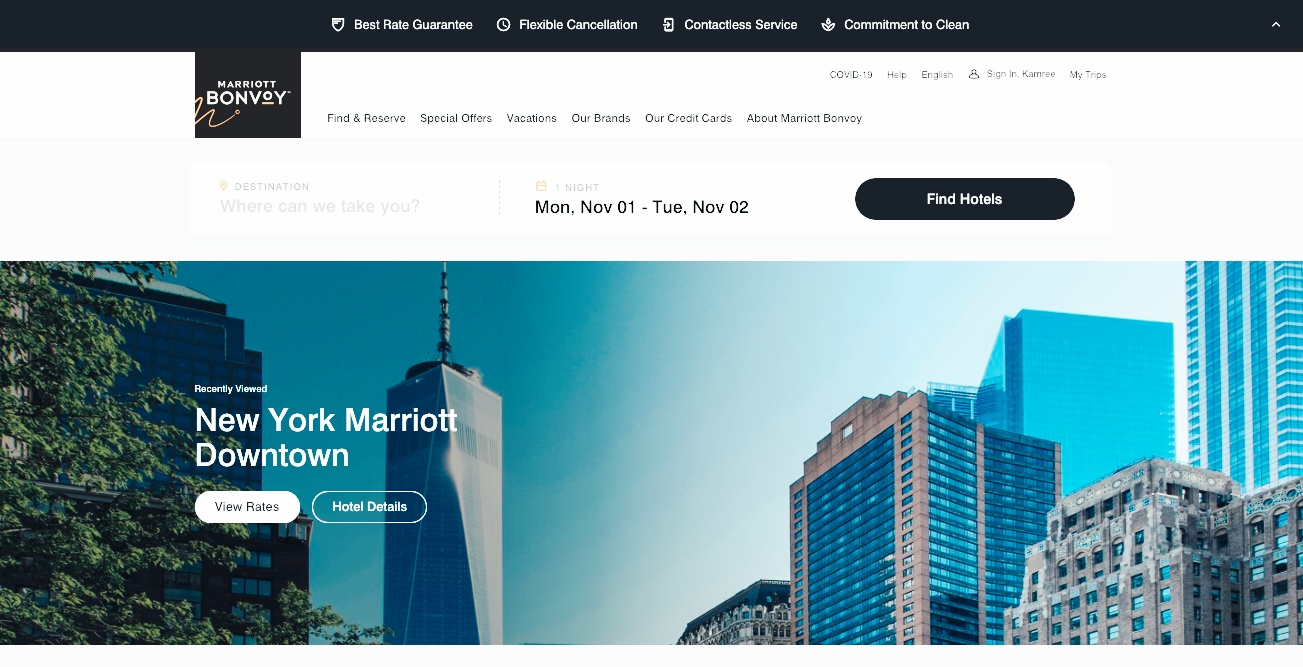This is an image showcasing the Marriott Hotel website for New York. The website features a predominantly white background with a sleek black and white color scheme. At the very top of the page, there's a slim black header with four options displayed in white text: "Best Rate Guarantee," "Flexible Cancellation," "Contactless Service," and "Commitment to Clean."

Beneath this header lies a white space containing several navigational options: "COVID-19," "Help," "English," "Sign In," and "My Trips," aligned from right to left. Just below, slightly to the left, are additional options including "Find & Reserve," "Special Offers," "Vacations," "Our Brands," "Our Credit Cards," and "About Marriott Bonvoy." To the left of these options, there's a small black square featuring the Marriott Bonvoy logo.

Underneath this section is another white bar, beginning with a destination input field labeled "Where can we take you?" This is followed by a reservation date selector showing "Monday, November 1st to Tuesday, November 2," indicating a one-night stay. Next to this is a prominent black button labeled "Find Hotels."

The background of the image reveals a serene cityscape featuring a few buildings, a green tree, and a blue sky. Overlaid on this is a smaller section with white text that reads "Recently Viewed: New York Marriott Downtown." Below this text, there are two buttons: "View Rates" and "Hotel Details."